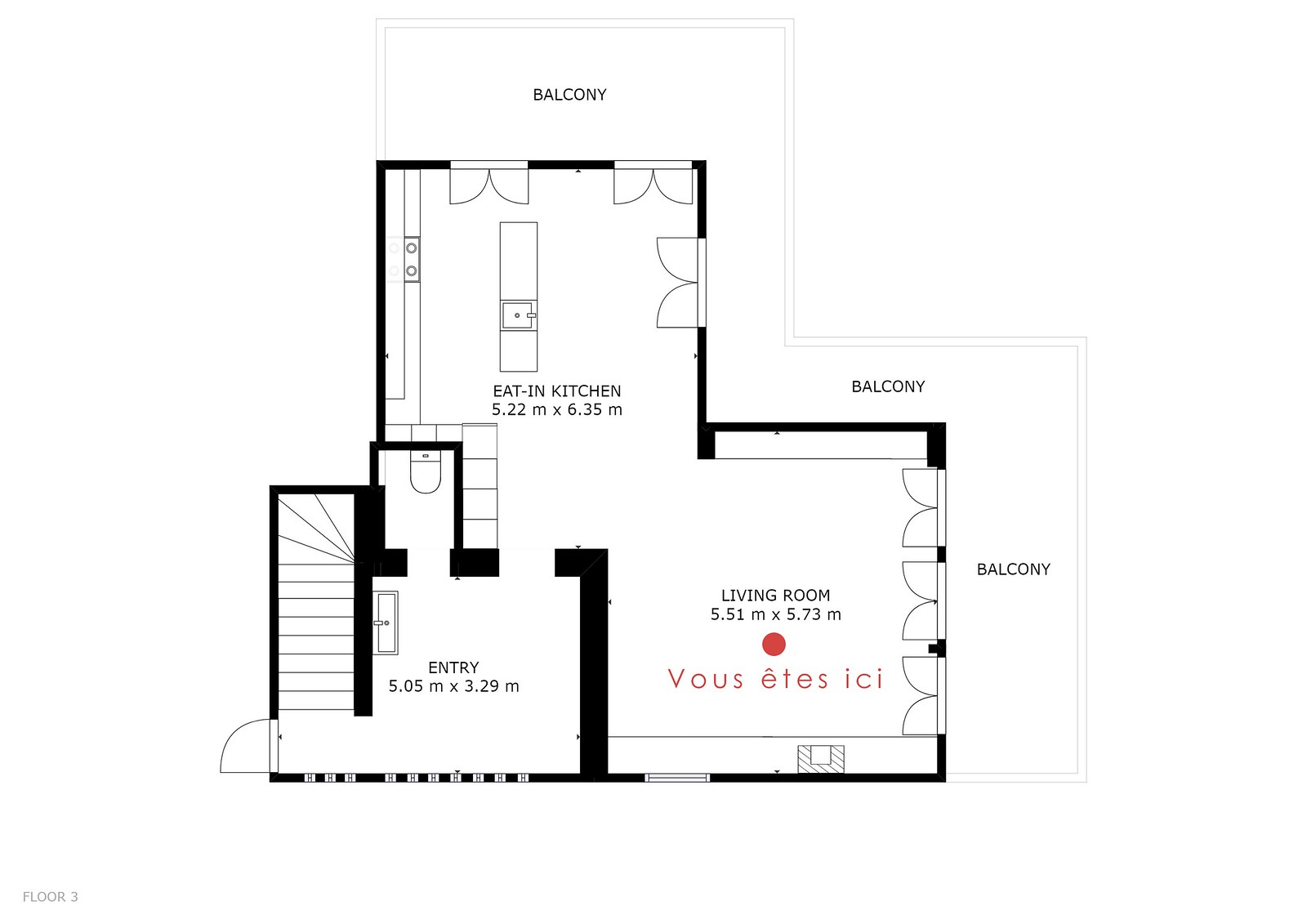This detailed floor plan represents the third floor of an apartment or house. In the bottom left corner, it is labeled "Floor 3." At the top of the layout, the word "Balcony" is prominently noted, indicating that the balcony extends around both the top and right sides of the building.

Directly beneath the balcony on the top side are two doors that provide access to an eat-in kitchen, which measures 5.22 meters by 6.35 meters. Adjacent to the kitchen on the bottom right is the L-shaped living room, with dimensions of 5.51 meters by 5.73 meters. The living room features three doors on its right side that also lead to the balcony, fully integrating the living space with the outdoor area and providing a seamless flow between the kitchen and the balcony.

To the left of the living room is an entryway measuring 5.05 meters by 3.29 meters, which serves as the welcoming area of the floor. Directly in front of the entryway, you will find a half bathroom, providing convenient facilities for residents and guests alike. On the far left side of the entryway, there are stairs and a door, possibly leading to other floors of the building. This carefully designed layout ensures functionality and easy access to various parts of the apartment while maximizing the use of space and providing ample connection with the outdoor balcony.